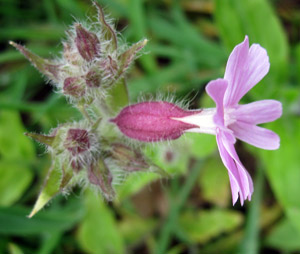This image captures a stunning, close-up view of a small orchid-colored flower opening to the right, displaying its beauty horizontally across the screen. The flower features four long, light purple to pink petals that flare out, and these petals emerge from a white stalk with a dark purple base. The center of the flower is white, and near this center, there is a larger dark purple bulb-like structure. At the base, the flower is surrounded by two fuzzy, spiky leaves—one positioned upwards and the other downwards—that are a mix of brown and green. The background, filled with green foliage and some grass, is artistically blurred to highlight the detailed focus on the flower and its unique structure.